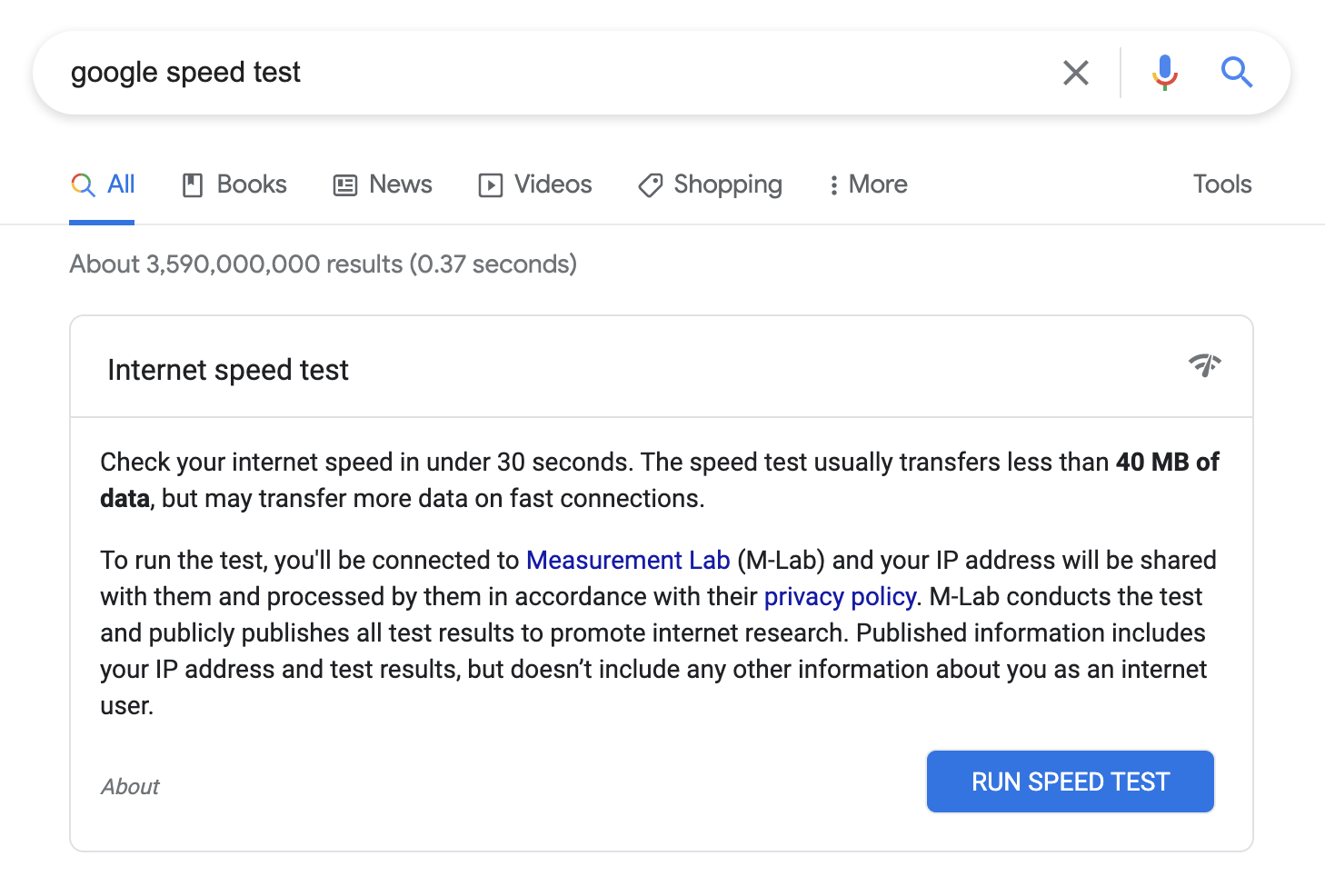The image is a screenshot of a Google search query for "Google speed test." At the top, the familiar Google search bar displays the entered query "Google speed test," with several navigational tabs beneath it, including "All," "Books," "News," "Videos," "Shopping," and a "More" dropdown menu, indicating additional options. Adjacent to these options is the "Tools" button on the far right.

In the lower right corner of the screen, the search results are shown, revealing a staggering 3,590,000,000 hits found in just 0.37 seconds. The top result is highlighted under the heading "Internet Speed Test," providing a brief description: "Check your internet speed in under 30 seconds. The speed test usually transfers less than 40 megabytes of data, but may transfer more data on fast connections."

The description further clarifies that to execute the test, users will connect to Measurement Lab (M-Lab), and their IP address will be shared and processed according to M-Lab's privacy policy. It notes that M-Lab will conduct the speed test and publicly publish all results to promote internet research. The published information will include the user's IP address and test results but will exclude any other personal data.

At the bottom of the description, a prominent blue button labeled "Run Speed Test" invites users to initiate the test.